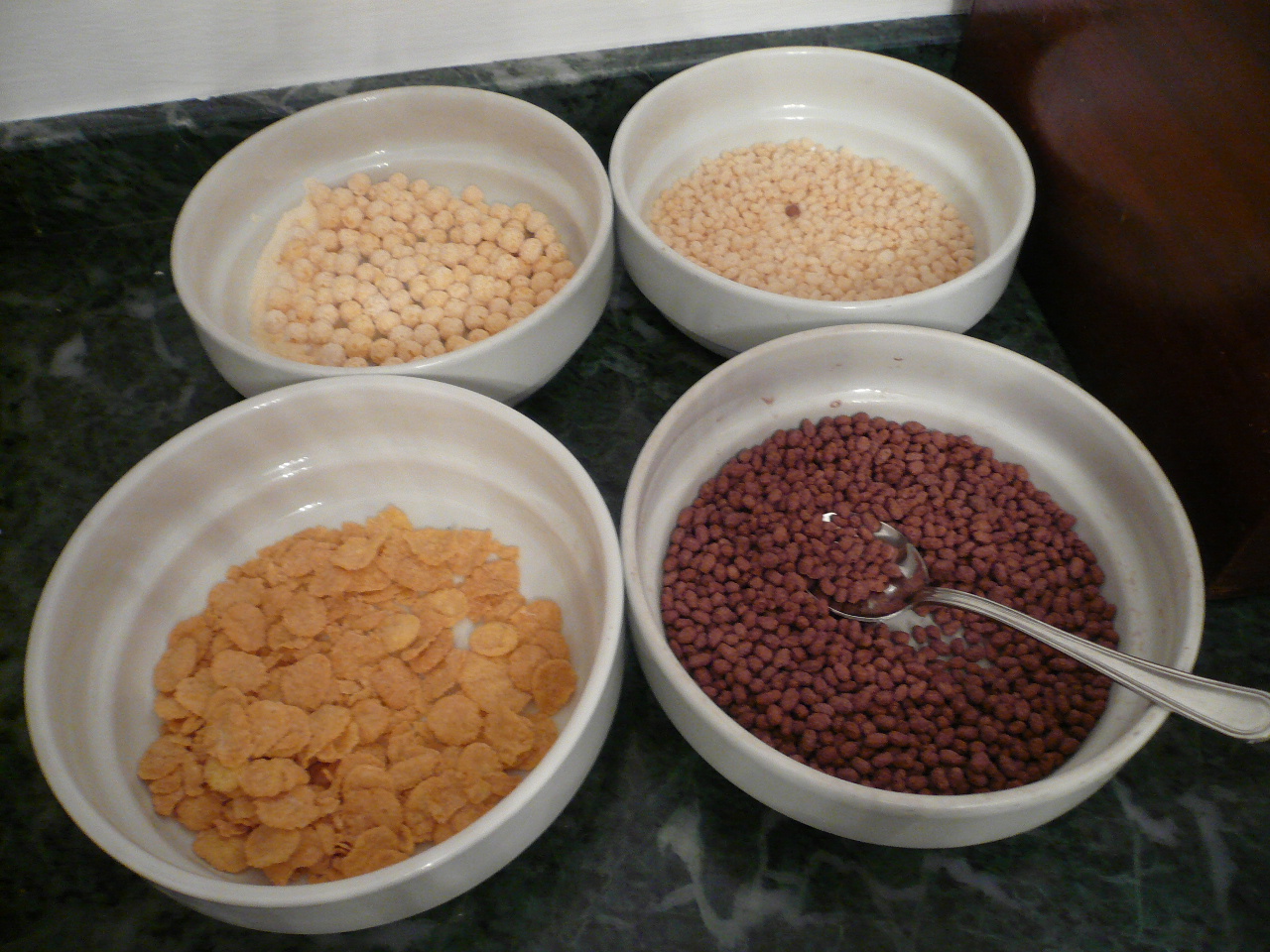In this detailed photograph, four white ceramic bowls filled with different kinds of dry breakfast cereals are displayed on a green marble countertop with a matching backsplash. The bowls are arranged in a two-by-two layout. The cereal types are as follows: the bowl at the top left contains medium-sized tan balls that resemble puffed cereal; the top right bowl holds small tan grains, similar to Rice Krispies; the bottom left bowl features light brown flakes, akin to cornflakes; and the bottom right bowl has small brown nuggets, likely cocoa-flavored puffed cereal. A silver spoon is placed in the bowl with the chocolate cereal. The background includes a white wall, providing a clean and neutral contrast to the vibrant cereals and rich countertop.